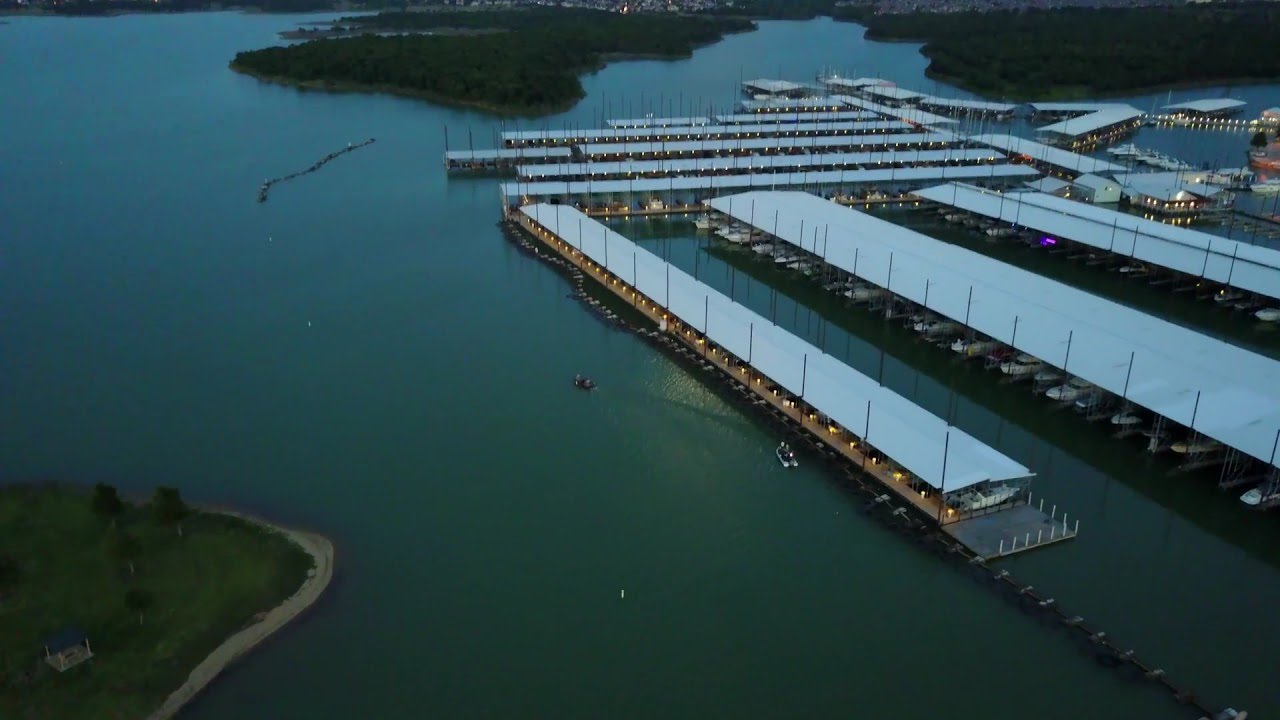This photograph, captured during the evening or early night, depicts an expansive, well-illuminated lake scene with numerous boating facilities. The central focus is on an array of long piers, extending into the water, each topped with gray or white roofs. These structures serve as boat storage or docking areas, housing multiple motorboats which are neatly parked underneath. The scene is intricately lit by numerous yellow lights, suggesting a well-maintained and upscale marina. Surrounding the docks are small, tree-covered islands and grassy areas, contributing to a serene, picturesque landscape. The water, a blue-green hue, reflects the glowing lights, heightening the tranquil yet sophisticated ambiance.